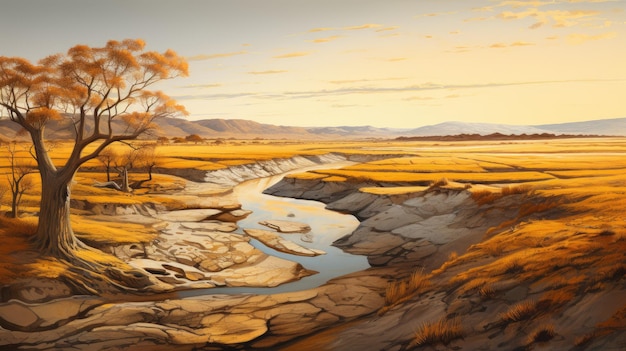This watercolor painting depicts a warm, golden-hued savannah landscape with a realistic touch. Dominating the left side of the composition, a large tree with clustered, golden-brown leaves and exposed roots stands adjacent to a meandering creek that cuts through rocky, stone-gray banks. The prairie-like flatlands stretch into the distance, glowing in rich orange and tan-brown tones, giving a sunset impression. In the far background, a full range of brown hills wraps around the scene, adding depth to the expansive vista. The sky, tinged with a gold hue and a blue tint on the left, is adorned with wispy, faded orange clouds, completing this vivid and atmospheric portrayal of a serene, sun-drenched wasteland.